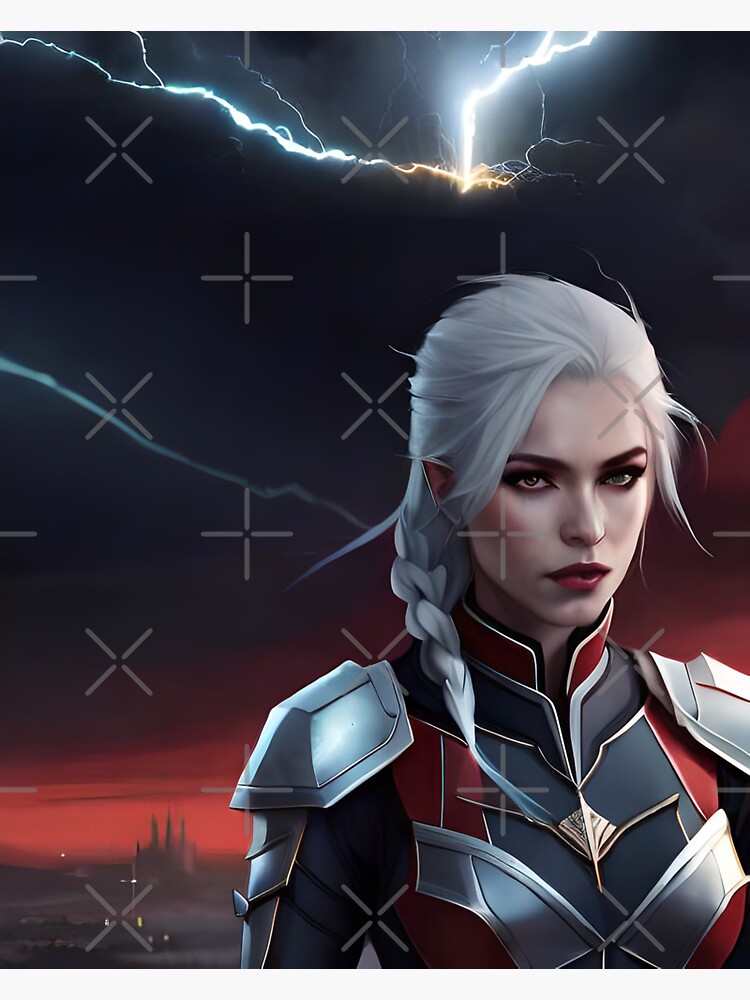The image depicts a highly detailed, artist's rendering of a female white knight with distinctive, elven-like pointed ears, set in a science fiction context. Her hair is a striking grayish-white, styled in a braid that drapes over her right shoulder and down her breast, almost wrapping around her neck. She's fair-skinned with dark outlines around her eyes and vibrant red lips, exuding a striking, almost otherworldly beauty. Her ornate armor is a mix of futuristic and medieval elements, featuring shoulder guards in silver, a decorative breastplate that transitions from silver to black and gold, and a red, gold-framed collar around her neck. The knight stands at the bottom right of the image, staring off to the side, amidst a dramatic background: a black sky crackling with lightning bolts, which fork and strike against each other, and a horizon lit by a scarlet sunset that fades from deep burgundy to lighter shades of red. In the distance, the spires and turrets of a castle-like structure silhouette against the vibrant sky. The ground beneath her feet is a somber gray, completing the scene with a stark, otherworldly ambiance reminiscent of a video game or digital artwork.